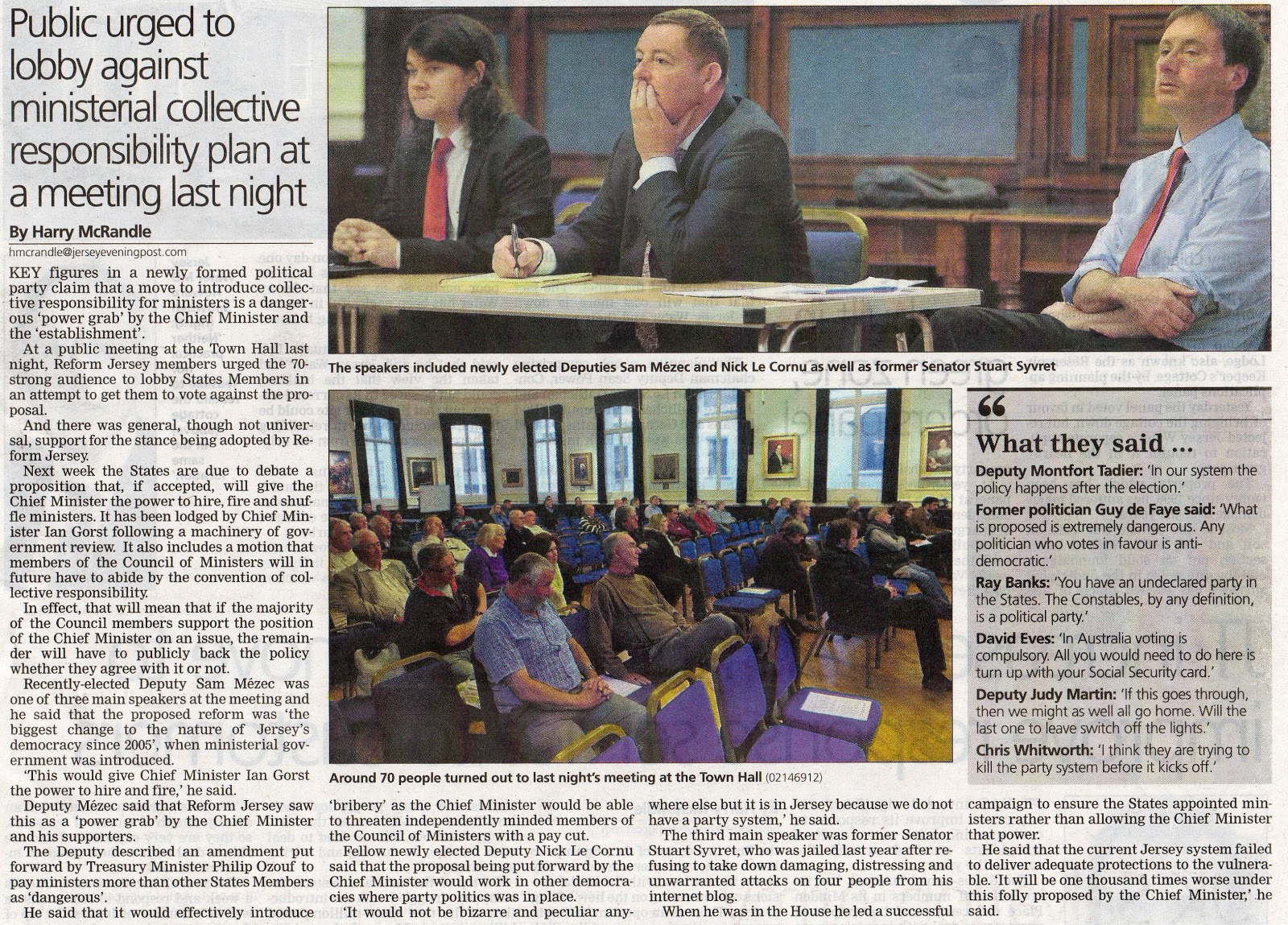A newspaper clipping features a headline in the upper left corner: "Public Urge to Lobby Against Ministerial Collective Responsibility Plan at Last Night’s Meeting," written by Harry McRandall in the largest type. The visual background is a gray, newspaper-colored print. 

The clipping includes two photos: one depicts three individuals, and the other shows an audience seated in blue chairs attentively listening. Under the first photo, the caption reads: "Speakers included newly elected deputies Sam Mazik and Nick LeCornu, as well as former Senator Stuart Sybert." These key figures in the newly formed political party argue that a proposed move to introduce collective responsibility for ministers is a dangerous power grab by the Chief Minister and the establishment.

During a public meeting at the Town Hall last night, Reform Jersey members encouraged the 70-strong audience to lobby States members to oppose the proposal. The room demonstrated general, though not universal, support for the stance adopted by Reform Jersey. 

Next week, the States are scheduled to debate the proposition which, if accepted, will grant the Chief Minister the authority to hire, fire, and shuffle ministers. The Reform Jersey members emphasized the importance of lobbying against what they perceive as an overreaching consolidation of power.